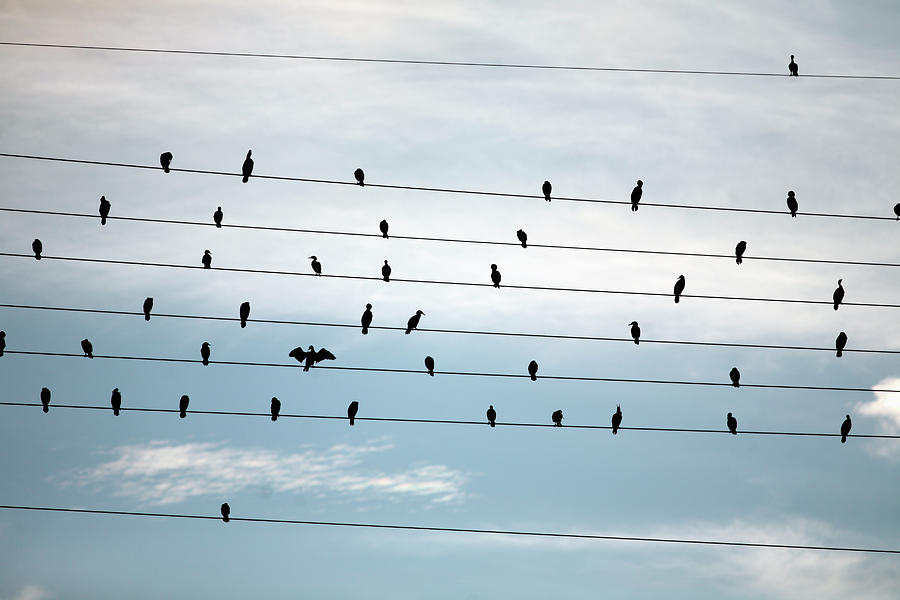The image depicts a wide, rectangular shot of a cloudy, bluish-gray sky, accentuated by numerous clouds concentrated more heavily at the top. Eight power lines stretch across the scene, each populated with numerous black birds. In total, 44 birds are scattered along these lines, sitting mostly in clusters. Notably, the topmost and bottom lines each have only one bird perched on them, while the others host several birds. Among them, one bird on the third line from the bottom stands out with its wings spread open, seemingly about to take flight. The birds are all shadowy black, creating a stark contrast against the brooding sky.